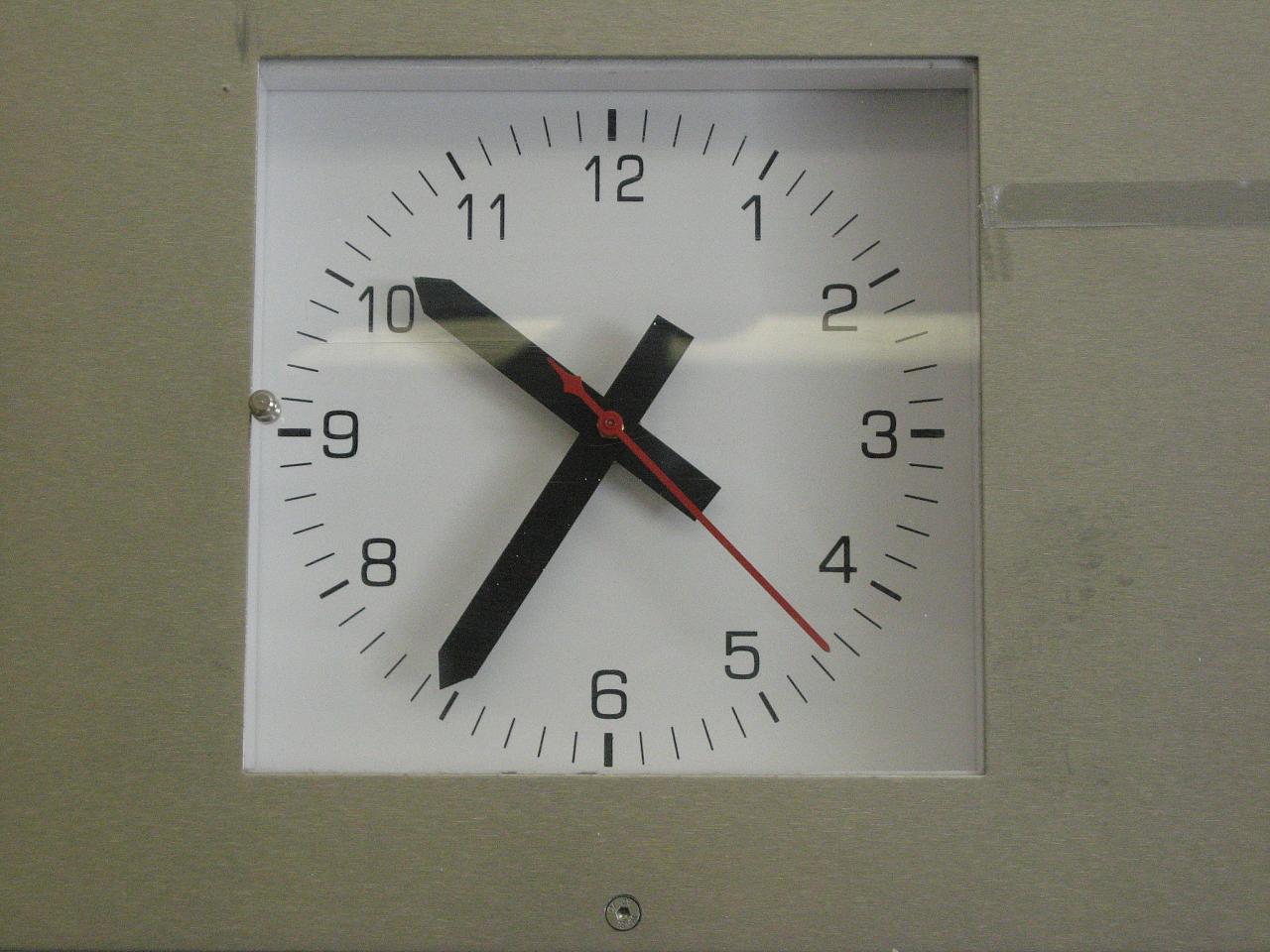This photograph features a centrally positioned square clock mounted on a beige-colored wall. The clock, encased in a white frame with a glass cover, displays distinct thick black hands for the hours and minutes, and a vibrant red second hand. The clock shows the time as a little after ten, with the minute hand covering the seven, and the second hand pointing between the four and five. Notably, there's a piece of tape extending from the clock to the edge of the image, located about one-fifth or one-quarter of the way down from the top right corner. Additionally, a small screw is visible at the bottom center of the frame, embedded in the wall.